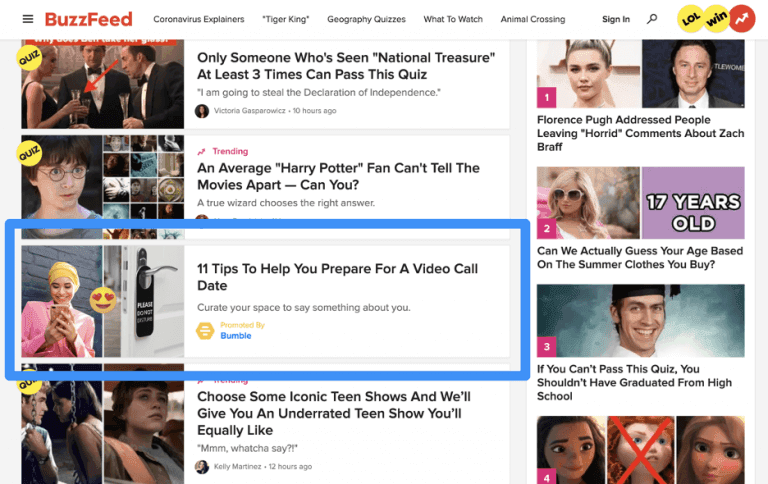The image features a predominantly white background with three black lines at the top, followed by the "BuzzFeed" logo in red. Below this, there are several blue links reading "Coronavirus Explainers," "Tiger King," "Geography Quizzes," "What to Watch," and "Animal Crossing," along with a "Sign In" option. Two yellow circles labeled "LOL" and "WIN" and a red circle with a small, crooked white arrow also appear near the top.

In the central section, a yellow box marked "Quiz" is positioned beside a red arrow pointing at a girl's drink. This section is captioned, "Only someone who's seen National Treasure at least three times can pass this quiz." Below it, a smaller text states, "I am going to steal the Declaration of Independence."

Further down, another yellow circle marked "Quiz" leads into a segment featuring Harry Potter. Several small images line the side, under the header "Trending" in pink. Adjacent to this is a section reading, "An average Harry Potter fan can't tell the movies apart, can you? A true wizard chooses the right answer."

Next, a blue-enclosed box features a photo of a girl with a smiley face and red heart eyes. This section is entitled "Eleven tips to help you prepare for a video call date," followed by the phrase "Curate your space to say something about you." Beside this is a little yellow hexagon labeled "Bumble."

In the concluding segment, there are two pictures beneath another yellow "Quiz" sign. The caption reads, "Choose some iconic teen shows, and we'll give you an underrated teen show you'll equally like," followed by the phrase "Hmm, what you say?" Next to these images are two additional pictures. The first features a girl within a pink box labeled "1," titled "Florence Pugh addressed people leaving horrid comments about Zach Braff." The second image shows another girl beside a pink "2" box, with the challenge "Can we actually guess your age based on the summer clothes you buy?" and "17 years old" in a purple box beside her. The third picture depicts a young man in a pink "3" box with the text, "If you can't pass this quiz, you shouldn’t have graduated from high school."

Finally, three doll pictures are displayed, with the middle one marked with a red “X” and labeled with the pink "4" box.